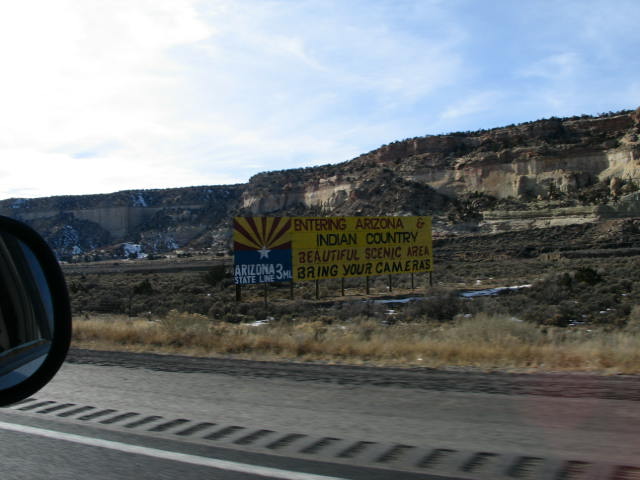This image, taken from a moving car's passenger side, captures a scenic Arizona landscape. A side view mirror on the far left indicates the photo was likely taken from the right side window. The foreground features a road with a white line and small bumps that serve as rumble strips, along with patches of gravel and grassy areas transitioning from tan to dark green.

The main focus is a billboard-style sign, supported by wooden posts, which vividly stands out against the desert backdrop. The primary section of the sign is orange with red and black lettering, stating: "Entering Arizona Indian Country" in bold red and black text at the top, followed by "Beautiful Scenic Area" in red, and "Bring Your Cameras" in black. Additionally, it announces "Arizona State Line - Three Miles" and includes elements reminiscent of the Arizona state flag.

In the background, there are majestic rock formations characteristic of canyon landscapes, featuring tall, flat-topped mountains with rocky edges. The sky above is a clear blue, slightly hazy, adding to the overall beauty of this roadside scene.